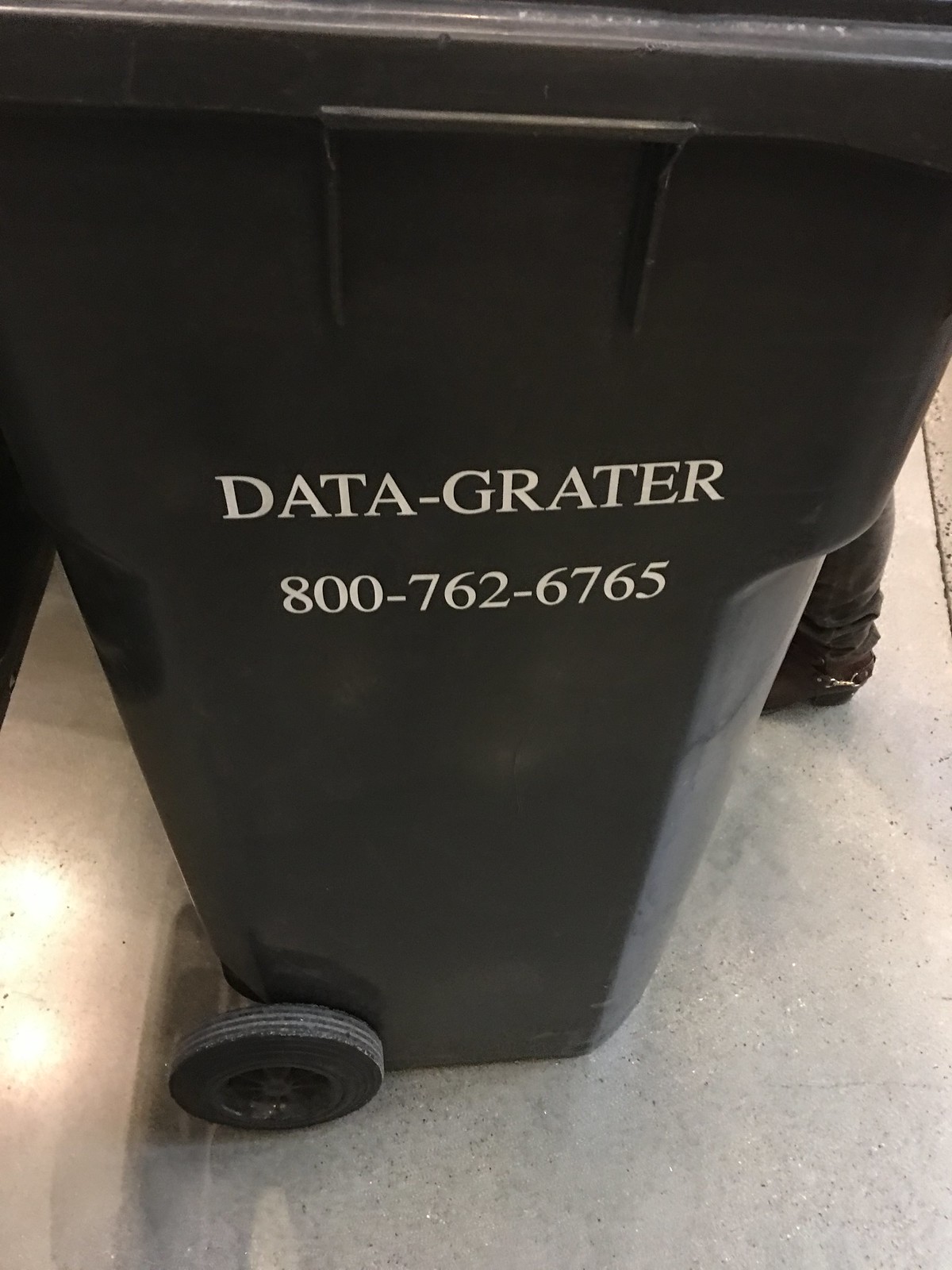This colour photograph, taken in portrait orientation, shows a black wheelie bin commonly found in the United Kingdom, viewed from a roughly 45-degree high angle. The wheelie bin appears well-used, with a slightly dirty wheel that exhibits a white, dirty-grey banding around its circumference. Prominently positioned in the middle of the side of the bin, there is text in white that reads "DATA-GRETER" followed by the phone number "800-762-6765." The bin is set on a concrete surface that shows cracks and imperfections. To the left of the wheelie bin, the concrete is overexposed, producing yellow, prominent reflections due to light sources. Additionally, there is a small strip of blacktop visible adjacent to the concrete. The photo effectively conveys the practical and utilitarian nature of the scene.